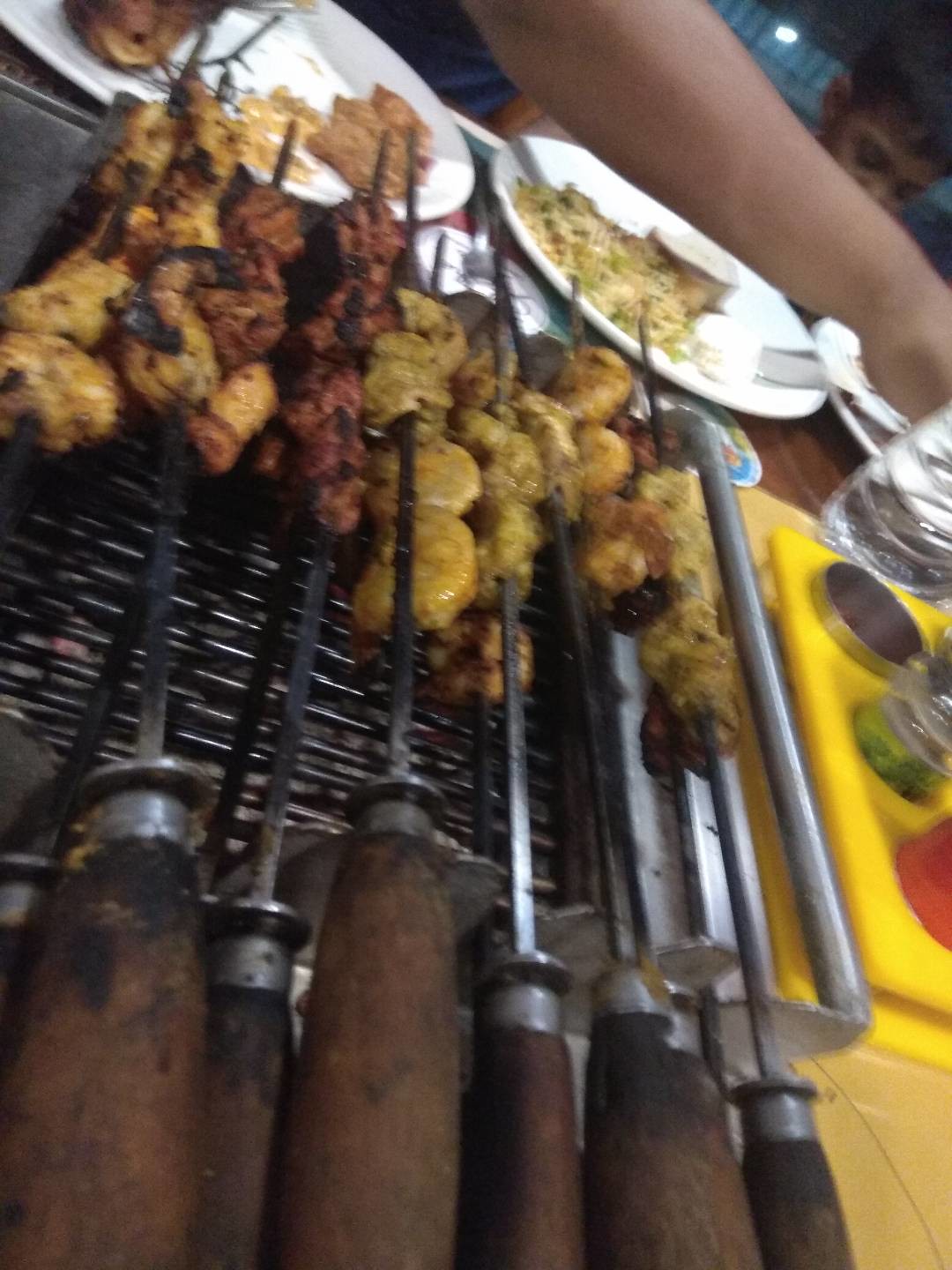The photograph captures a dining table at a restaurant, featuring a metal hibachi-style grill at its center, filled with a variety of skewers or shish kebabs. The skewers appear to contain chunks of meat, possibly chicken, beef, and shrimp, with some pieces more charred and browned than others, illustrating a range of cooking times and meat types. The skewers have brown handles, and they stretch across the grill. At the far end of the table, two white plates are visible, with indistinct food items on them, likely due to the picture's quality, possibly rice. A person's arm is extended across the table, reaching for an item on the right side of the image, which includes a yellow object that looks like a condiment holder, as well as a bottle of water. The overall scene suggests an active dining experience with shared plates and mixed textures and colors of food.